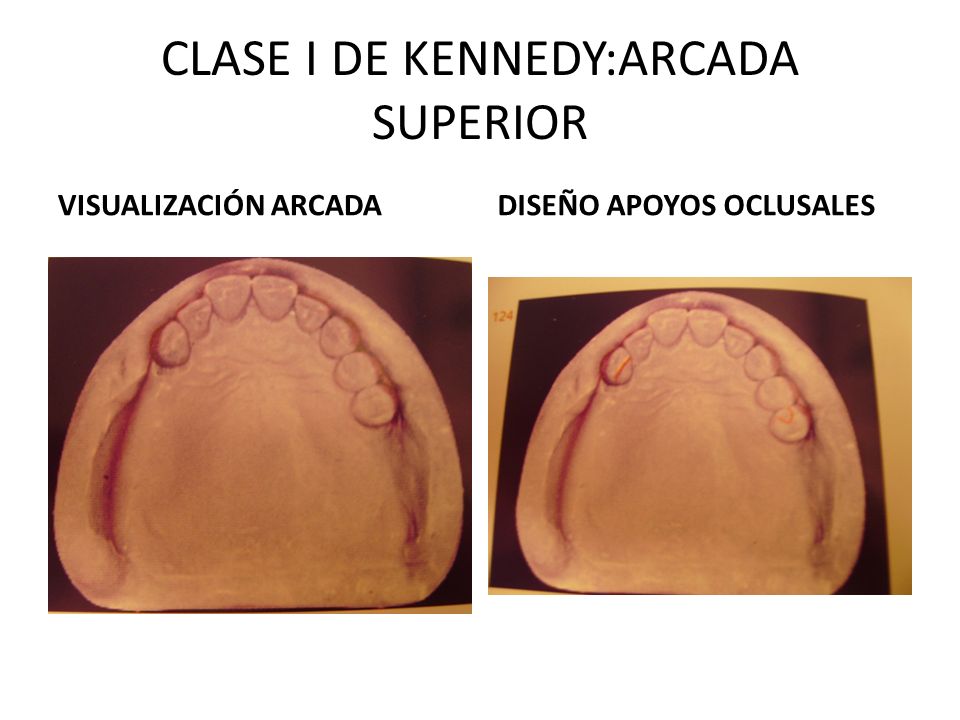The image appears to be an educational slide likely used in a dental school setting. The slide features a plain white background with prominent black capital letters stating the title "CLASE I DE KENNEDY: ARCADA SUPERIOR." Below the title, there are two labeled dental images presented side by side. 

The left image is labeled "Visualización Arcada," while the right image is labeled "Diseño Apoyos Oclusales." Both images show a top view of a dental mold or impression of a jaw, featuring multiple missing teeth. The left image provides a closer, more detailed view, whereas the right image is slightly zoomed out. Notably, the right image displays an orange mark on the front-most left tooth, which is absent in the left image.

The images seem to depict different stages or aspects of studying dental arches, potentially for understanding the structural layout or planning for dental support elements. These materials are designed to aid students in visualizing and analyzing dental conditions. The background includes various rounds and pages, which do not contribute specific reference points but serve as a neutral backdrop for the primary visual information.